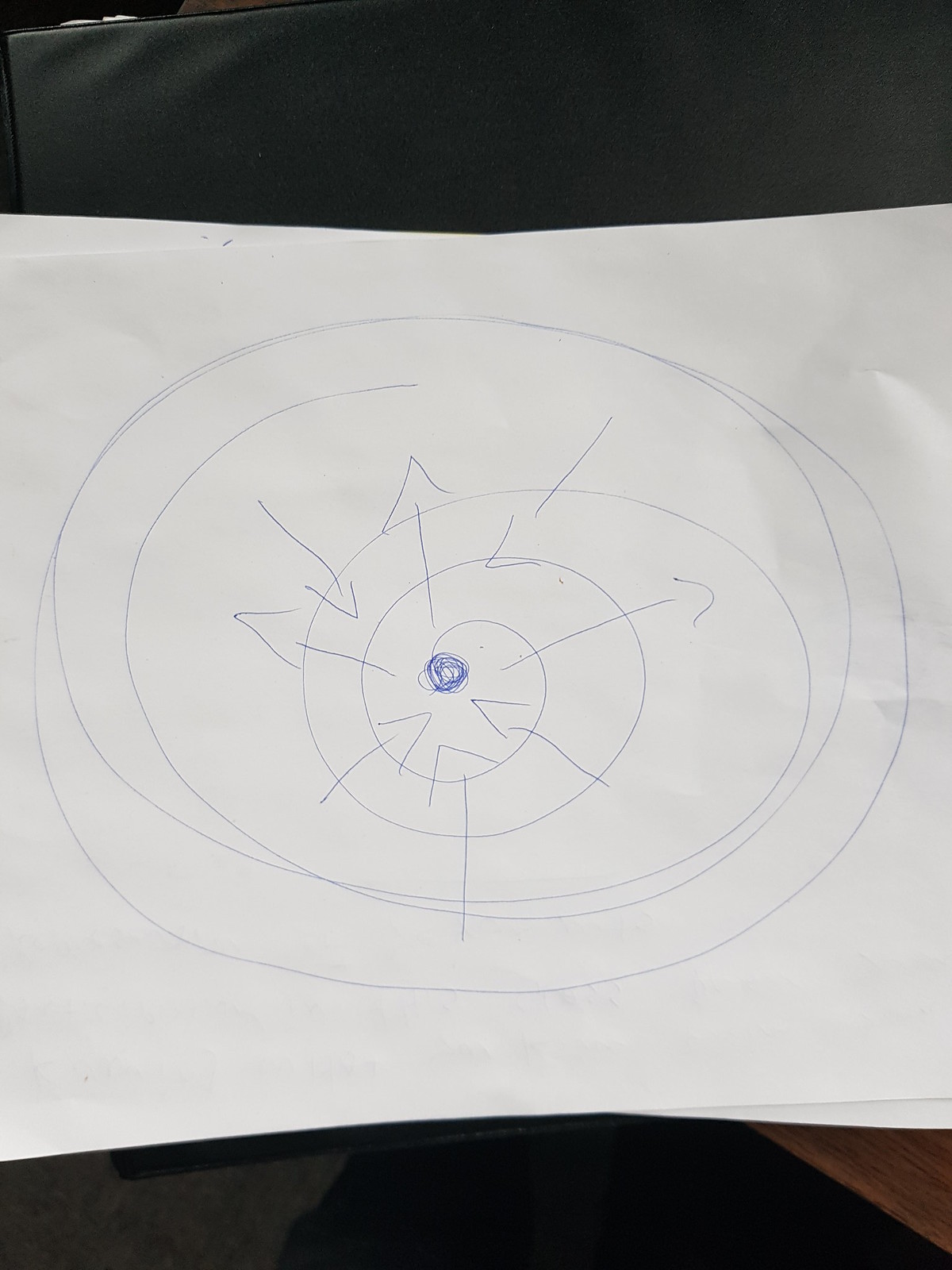A photograph captures a detailed blue ballpoint pen drawing on white paper. The centerpiece of the artwork is a densely filled circle, created with numerous ink swirls, serving as a focal point. Radiating from this central dot, a large counterclockwise spiral extends outward, almost filling the entire paper with its meticulous loops and curves. Emerging from the solid blue center, several lines with arrowheads are drawn, some pointing inward towards the center and others pointing outward, creating a dynamic visual interplay of direction and movement. The background is dark, with the faint impression of a wooden table supporting the paper, adding a subtle contrast to the bright, intricate drawing. No text is present on the drawing, allowing the viewer to focus entirely on the mesmerizing spiral and its directional elements.